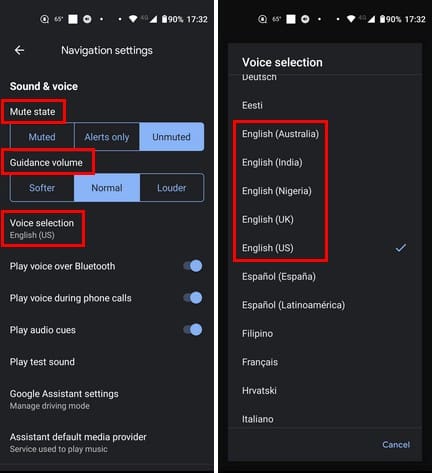The image features two screenshots from a navigation app's settings, specifically under the 'Sound and Voice' section.

**Left Screenshot:**
- The 'Muted State' option is highlighted in red, currently set to 'Unmuted'. Other available options include 'Muted' and 'Alerts Only'.
- The 'Guidance Volume' setting is also circled in red, with 'Normal' currently selected. Alternate volume levels available are 'Softer' and 'Louder'.
- The 'Voice Selection' is similarly highlighted in red, with the current setting being 'English (USA)'.

**Right Screenshot:**
- Displays the 'Voice Selection' menu, showing various language options:
  * 'English (Australia)'
  * 'English (India)'
  * 'English (Nigeria)'
  * 'English (UK)'
  * 'English (USA)' (currently selected)
  * Additional languages such as Dutch, Español (España), Español (Latin America), Filipino, Français, and Italiano are also listed.
  
Both screenshots include indicators for battery status and the current time, which is 17:19 (5:19 PM). This composite image is likely showcasing how users can adjust various audio settings within the app, including muting options, guidance volume, and language selection.